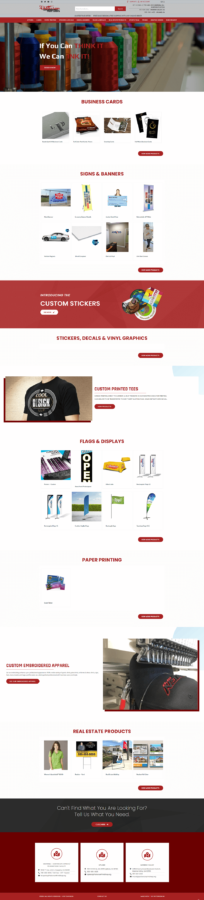**Descriptive Caption:**

The image appears to be a vertically extensive screenshot of a store's website, showcasing various promotional categories and products. At the very top, there's a slightly blurry banner with the tagline "If you can think it, we can sink it," where "think it" and "sink it" are highlighted in red text, while "if you can" and "we can" are in white. The backdrop of this text seems to be a shelf laden with items that resemble Legos.

Just below the banner, the section titled "Business Cards" is visible, accompanied by four small square images. Following this, the text "Banners" in bold red font appears with a series of eight smaller image boxes underneath. Further down, there is a prominent red rectangular banner with "Custom Stickers" written in white text, alongside an illustrative image positioned to its right. Continuing down the page, the categories "Stickers, Decals, and Vinyl Graphics" are listed in red writing, adjacent to a rectangular image displaying a person wearing a black shirt. Finally, at the very bottom of the image, there are three white boxes each featuring a red logo, completing the screenshot.